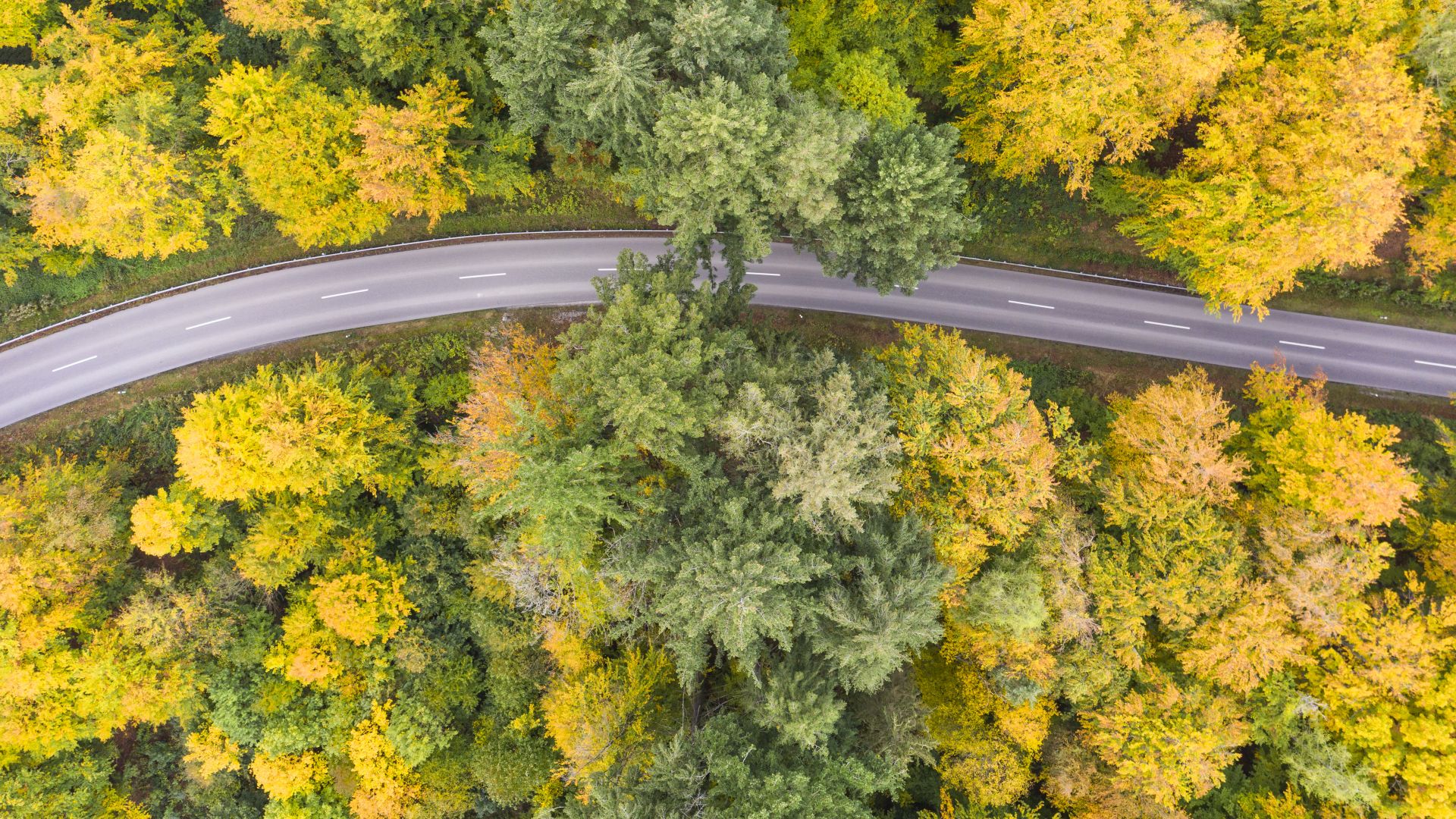This daytime aerial photograph captures a winding two-lane highway, characterized by its gray concrete surface and long white dashes that mark the lanes. The road curves gracefully around a mountainous area lush with trees. Bright green pine trees stand prominently in the middle of the scene, while the majority of the surrounding trees display varying shades of yellow and brown, signaling the onset of fall. Grass is visible at the base of the trees, which extend far down and ascend high into the landscape. The rural area depicted is devoid of cars, emphasizing the tranquil, undisturbed nature of the setting. The sun is clearly visible over the scene, enhancing the vivid contrast between the green and yellow foliage.